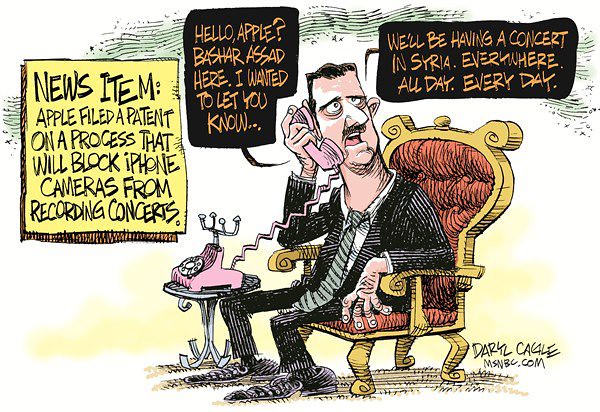In this politically charged cartoon by Daryl Cagle featured on msnbc.com, the focal point is a caricature of Syrian President Bashar al-Assad. He is depicted with exaggerated, elongated features, including a shovel-shaped head, exhausted eyes, minimal brown hair, and a brown mustache. He wears a pinstripe suit, striped tie, and sneakers, and sits in a regal-looking chair with red cushions and gold detailing, evoking a sense of false grandeur. At his ear is an old-fashioned pink landline phone. A yellow text box on the left of the cartoon announces, "News item: Apple filed a patent on a process that will block iPhone cameras from recording concerts." Assad’s speech bubbles, black with orange text, convey a satirical message: "Hello, Apple, Bashar Assad here. I wanted to let you know we'll be having a concert in Syria everywhere, all day, every day." The artist's name, Daryl Cagle, appears at the bottom right, alongside msnbc.com, grounding the piece in contemporary commentary.